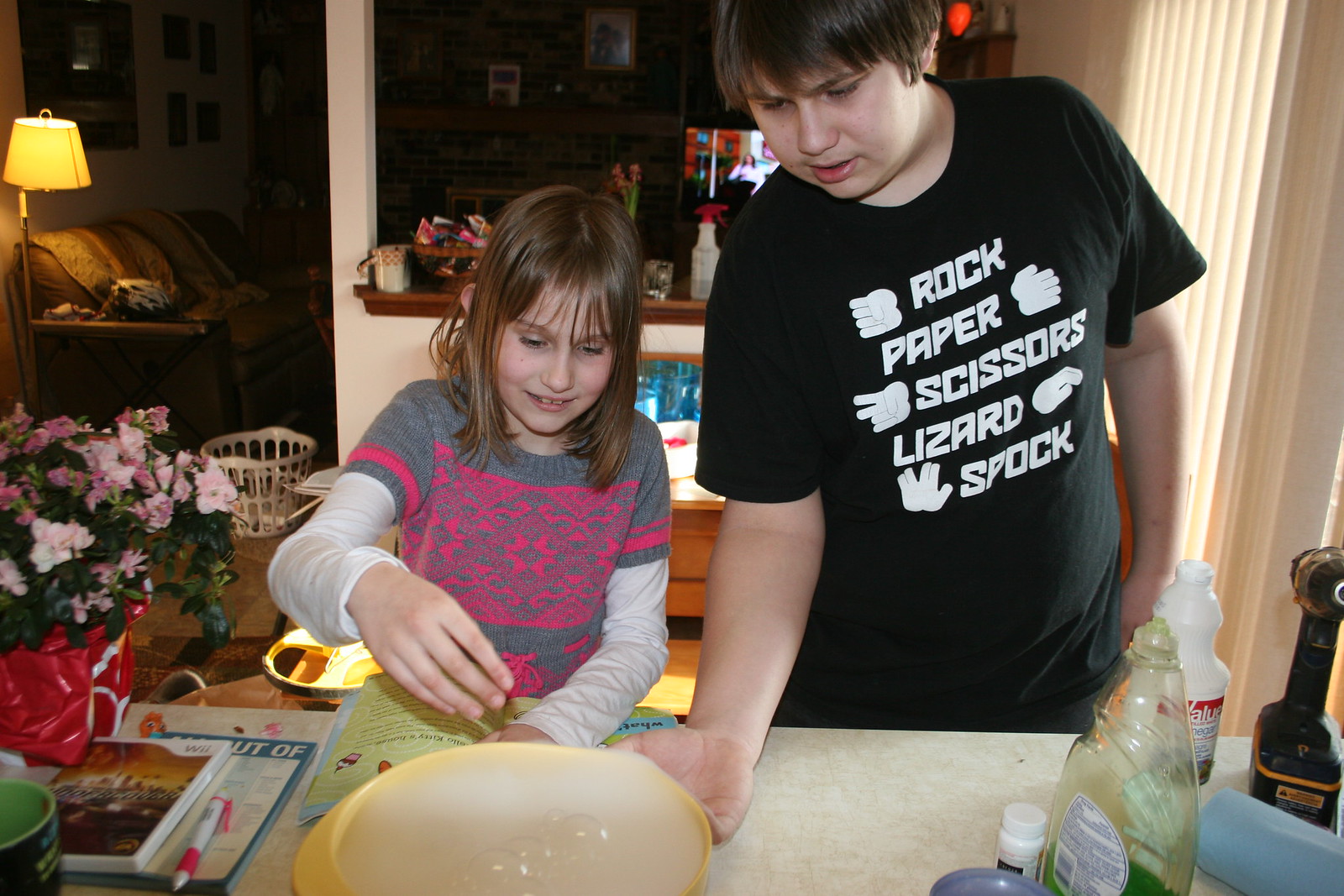In this indoor scene, a young girl and boy are engaged in an activity at a kitchen table, suggesting they're either cooking or conducting a science experiment. The girl, around 7 or 8 years old, blonde and dressed in a pink and gray sweater over a white long-sleeve shirt, is holding a book that appears to be a recipe. The boy, slightly older at about 9 or 10, is wearing a black shirt with the text "Rock, Paper, Scissors, Lizard, Spock" and is holding a bowl. The table they're working at is adorned with a red vase filled with flowers and flanked by various other not easily identifiable items, possibly including magazines and detergent bottles. The home's cozy atmosphere is highlighted by a lamp and a couch visible in the background, with several pictures on a mantle and a TV reflected in a mirror. The setting appears warm and familial, filled with different personal touches like flowers and assorted household items.